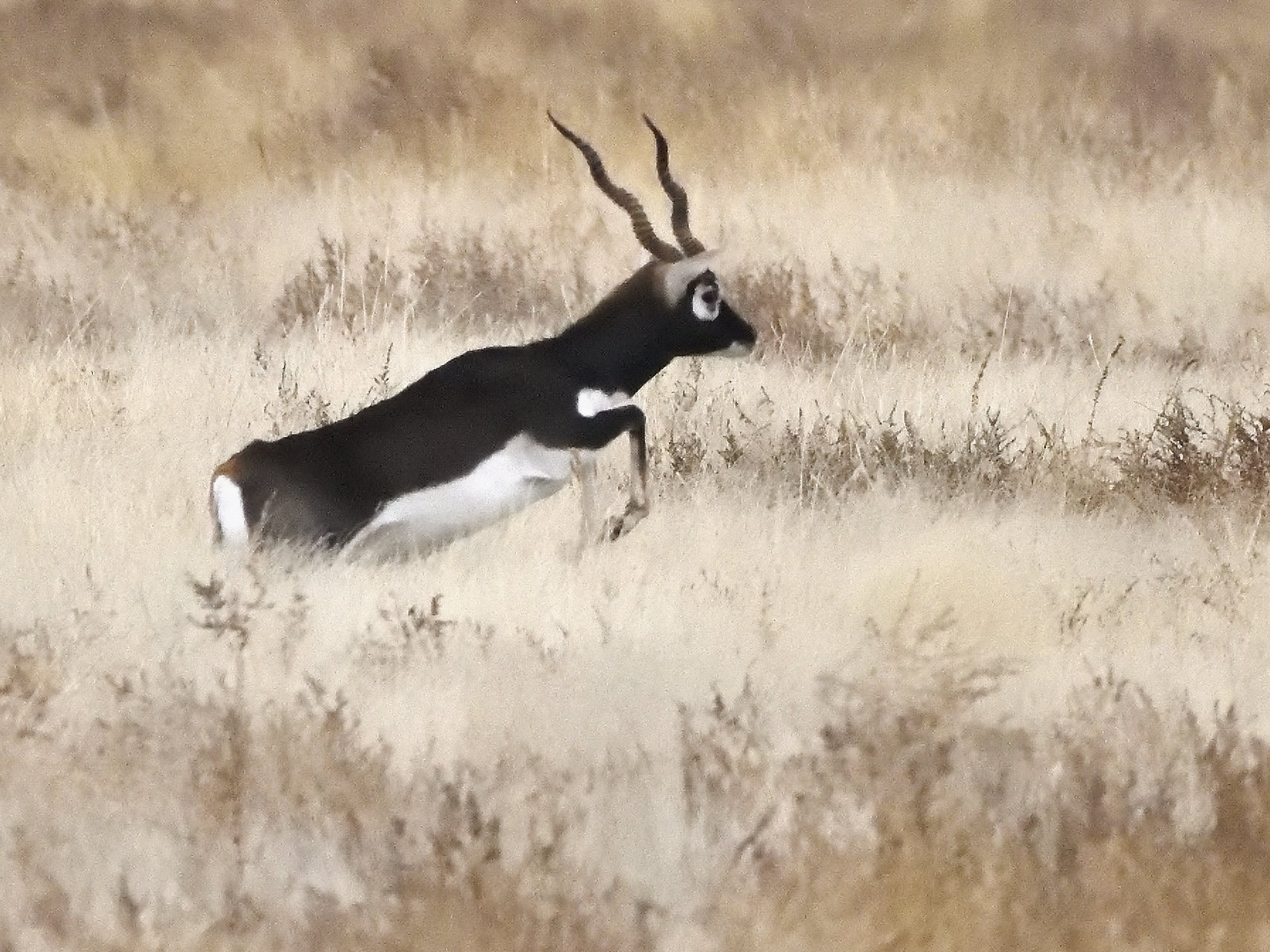The image captures an artistic color print, likely a painting, characterized by a strictly brown and white palette. The scene unfolds in a field of tall, dehydrated brown grass, emphasizing a natural yet desolate atmosphere. At the center, a brown and white antelope commands attention, its body predominantly brown with white accents on its chest, belly, and tail. The animal's most striking features include its long, wavy horns and the distinct white swatches around its eyes, including a pronounced circle above the eye. The antelope appears to be in motion, slightly leaping as if caught mid-gallop, suggesting agility and speed against the backdrop of the withered grass. Every element in the image—from the antelope's dynamic posture to the dried grasses—comes together to create a vibrant yet austere depiction of nature.